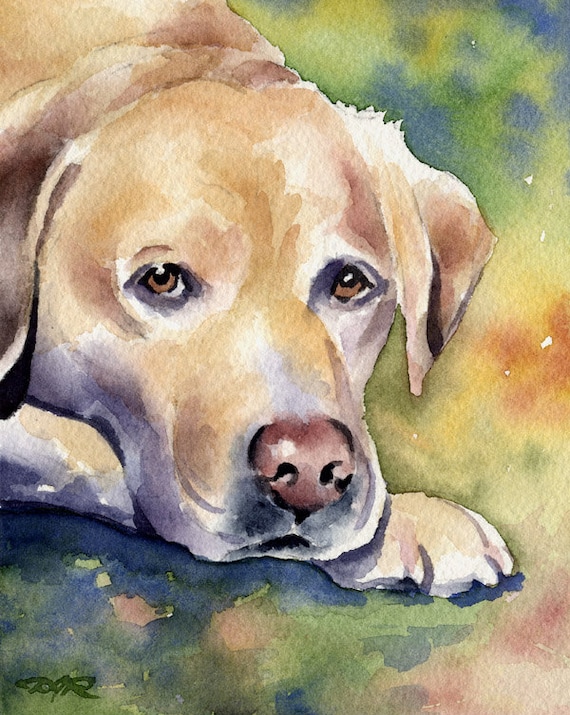This image is a detailed and vibrant color illustration created on watercolor paper. The painting medium appears to be either watercolor or gouache, characterized by its rich and blended hues. The subject of the illustration is a golden retriever, depicted with its head, back of the neck, and right paw visible, emerging from the top left corner of the frame. The dog is sitting and facing the viewer, looking slightly downward with its closed mouth and soulful brown eyes.

The artist has skillfully employed a palette of purples, browns, and yellows to capture the intricate details of the retriever's face through a series of washes. These colors blend seamlessly, giving depth and texture to the fur, and accentuating the dog's serene expression. The dog's nose features a delicate pink shading, adding an extra touch of realism and charm to the portrait.

The background is a harmonious wash of green, blue, yellow, and orange, which complements the warmer tones of the retriever and helps the figure stand out. This abstract backdrop provides a soft contrast through tonal variations, enhancing the focus on the dog's face and paws. Overall, the combination of thoughtful color choices and fluid brushstrokes culminates in a captivating and picturesque watercolor portrait of the golden retriever.